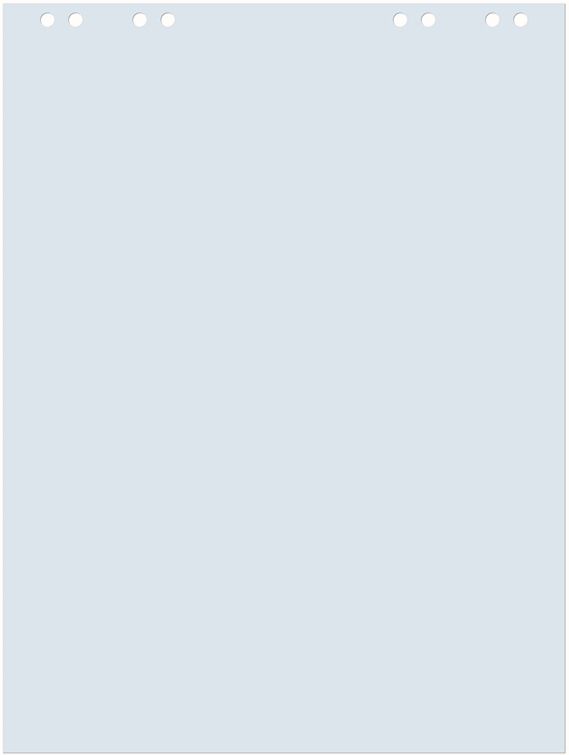The image appears to showcase a digital representation of a notepad or document. The background is entirely gray, evoking the look of a gray piece of paper. Along the top edge, there are evenly spaced dots resembling punch holes, suggesting that the paper could be part of a binder or notebook. The dots run across the top in a sequence, emphasizing the row of punch holes. The overall design is minimalist, with the gray expanse dominating the visual space, interrupted only by the consistent pattern of perforated holes at the top.